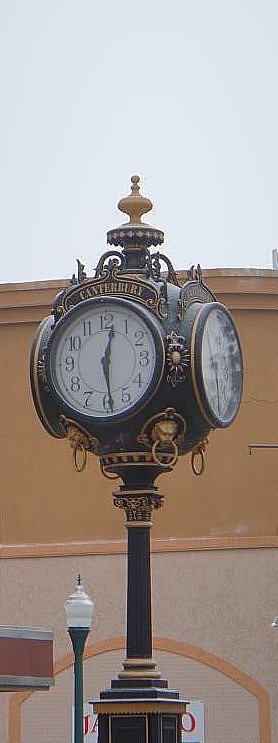The image features an ornate, old-fashioned clock fixture with four round, matching clock faces pointing in each cardinal direction, each showing the time at 12:29. The elaborate black metal frame, adorned with brown accents and lion heads, holds the identical white clock faces with black numbers and hands. The structure is globe-like, with a small gold-colored bulb at the top, sitting atop a black rod attached to a dark column. Directly behind the clock, a white board with partially visible red letters "JA" on the left and an "O" on the right can be seen. The setting includes an old-fashioned streetlight and a tan and brown building with an architectural dome reminiscent of Byzantine or Eastern designs. The entire scene exudes a vintage charm, hinting at an old European locale, possibly bearing the name "Canterbury" above each clock face.